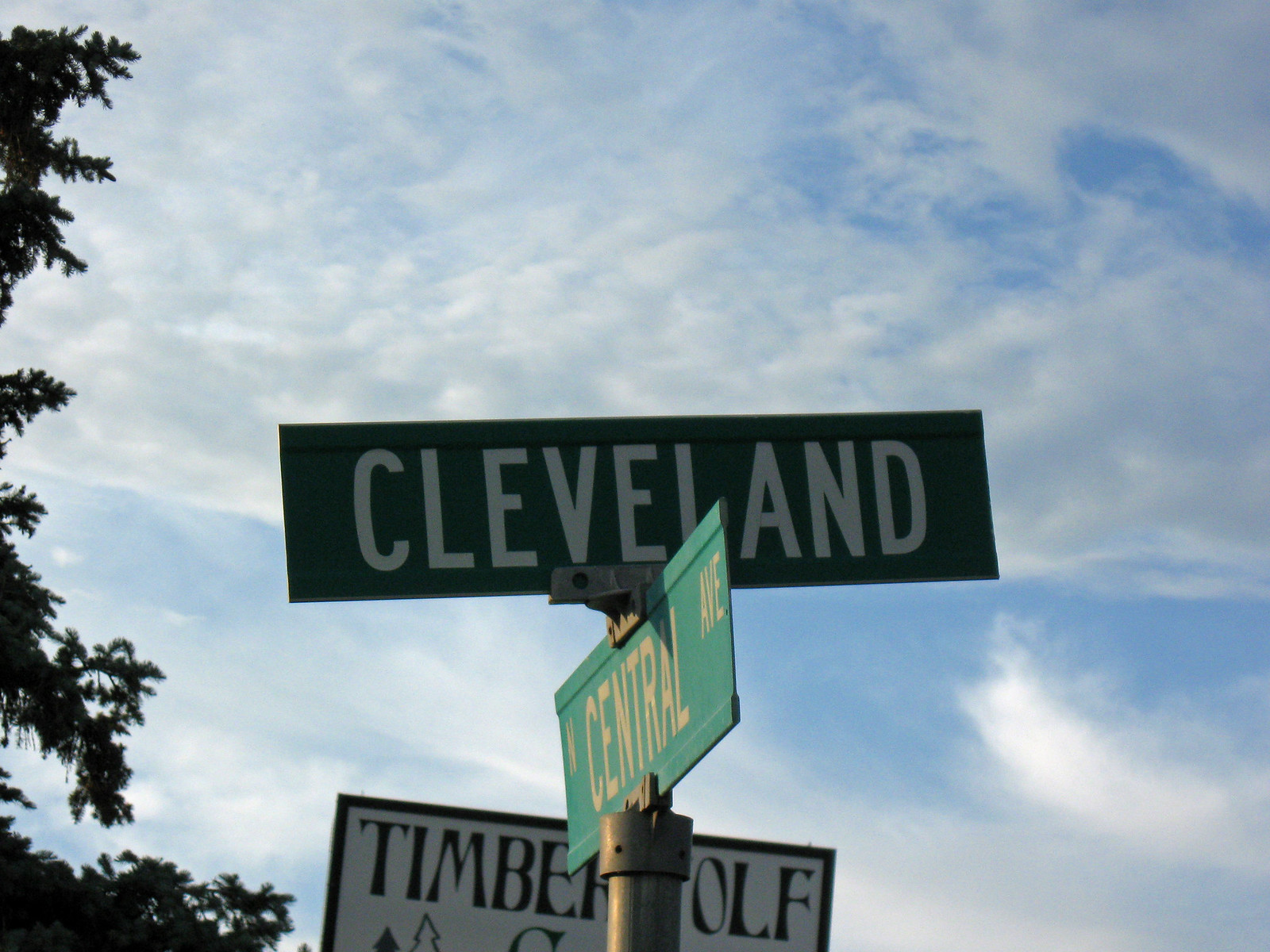This photograph captures a street intersection where Central Avenue meets Cleveland Street, depicted through long, green street signs with crisp white text. The image is taken almost parallel to Central Avenue, providing a clear view of the intersections' signage. At the top, "Cleveland" is clearly visible in bold white letters. Behind the main street signs, there is a secondary white sign with black text that partially reads "Timber Wolf," held up by a sturdy metal pole. This auxiliary sign features a black outline and some additional text cropped out at the bottom. In the left background, a dark evergreen tree stands tall, adding depth to the scene. The sky above is a vibrant blue, dotted with bright white clouds, suggesting a day with partial cloud cover.